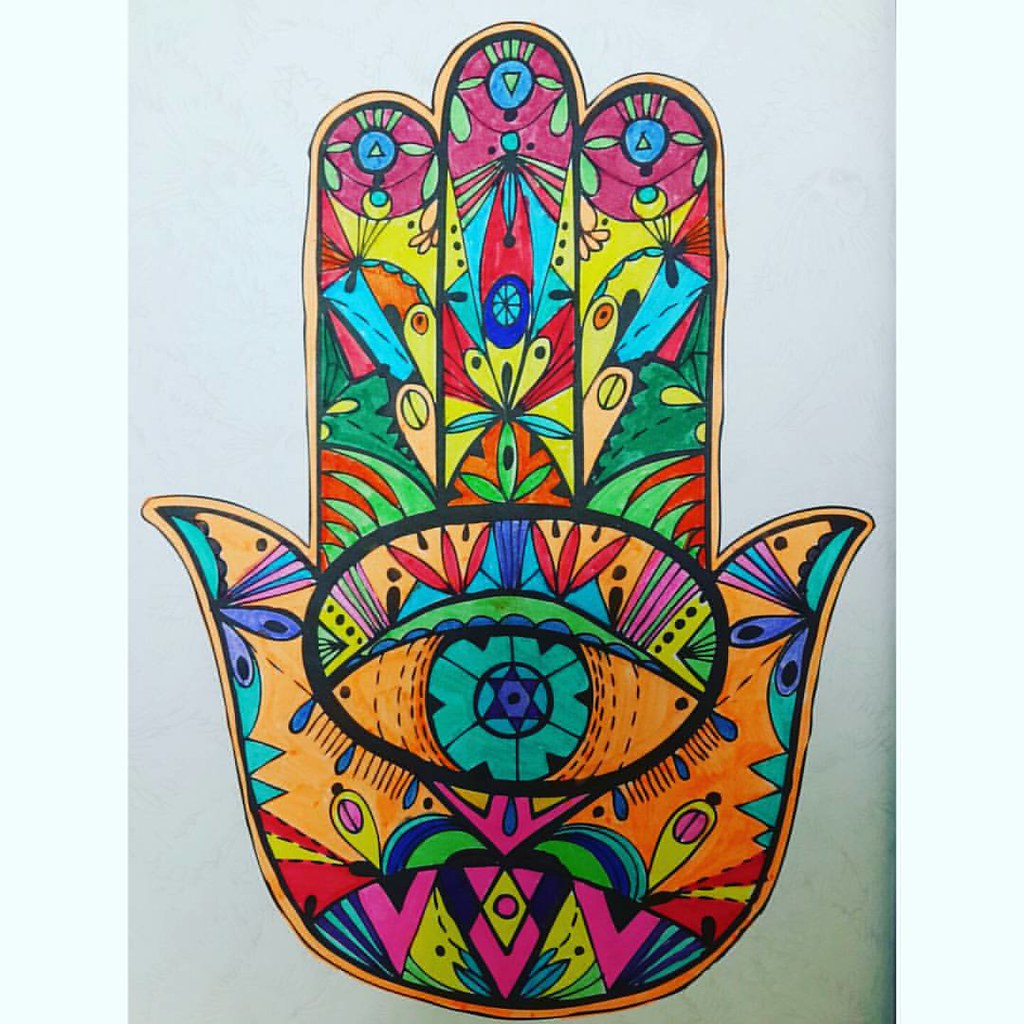This photograph showcases an intricately colored-in symbol of a Hamsa hand, featuring a prominent eye at its center. The Hamsa hand consists of three central fingers standing upright, flanked by pointed edges on both the left and right sides. A thick, black oval in the center flawlessly represents the eye. Each section of the symbol is meticulously outlined in dark black, encased in a thin orange border, followed by another slender black border. Within these outlines, vibrant designs reminiscent of a coloring book come to life, featuring an array of bright colors including orange, red, pink, green, turquoise, blue, and purple. The interior of the hand is adorned with various intricate patterns such as triangles, spirals, circles, and other geometric shapes, creating a visually captivating and detailed representation of this symbolic hand.